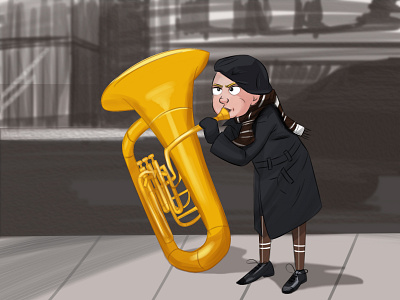This cartoon-like drawing vividly depicts a woman playing a disproportionately large tuba, which is as tall as she is and prominently placed at the center of the image. The tuba, painted a vibrant yellow, captures immediate attention. Positioned to the right of the tuba, the woman, with puffed-up cheeks signaling she's blowing into the mouthpiece, appears visibly angry. She is dressed warmly in a black coat, matching black hat, and a striped black-and-white scarf. Completing her ensemble are brown pants and black shoes. The scene is set outdoors, with the woman standing firmly on a gray sidewalk. Her shadow is clearly visible on the pavement, contributing to the depth of the scene. In the background, a blurred gray building with a few outlined windows on the left side provides a sense of urban environment. This detailed illustration combines elements of exaggeration and emotion, creating a striking and memorable visual.